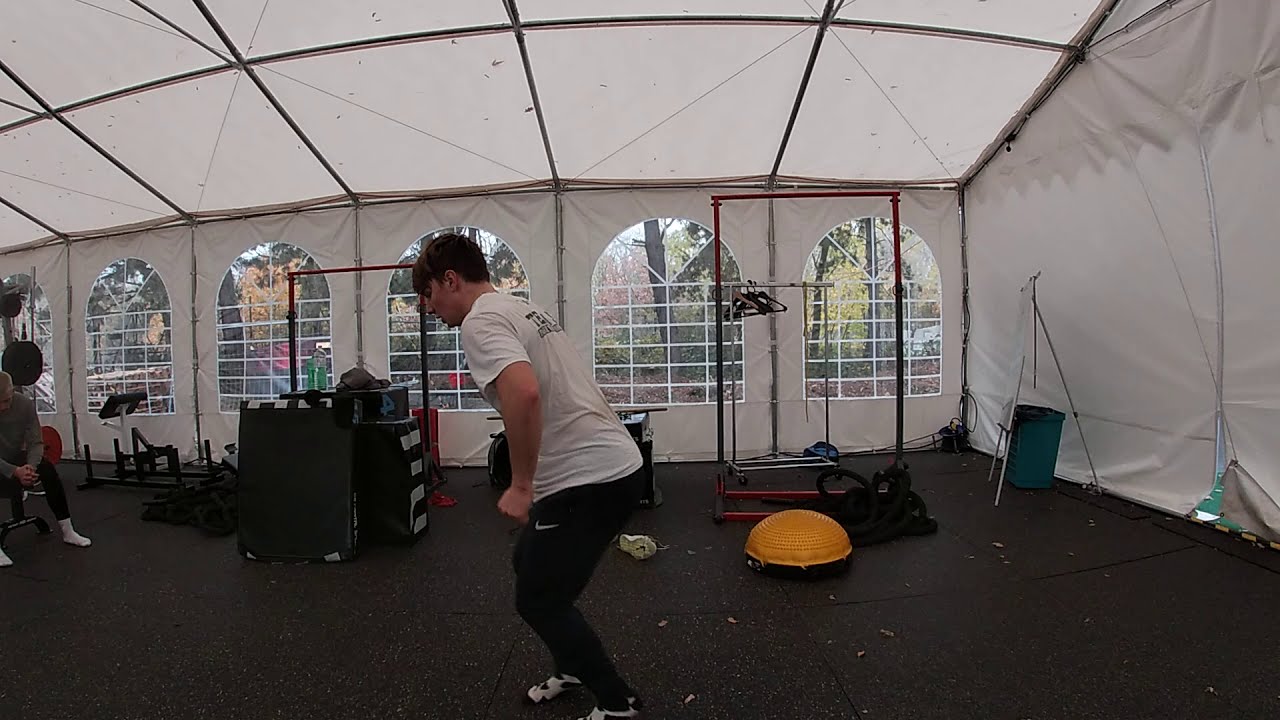The image is a landscape-oriented color photograph depicting a dynamic scene inside a white canvas tent structure that serves as a makeshift gym. At the center, a young man, captured in motion, appears to be either jumping or lunging forward, causing a slight blur in his figure which conveys his action. He is positioned with his body turned towards the left side of the image, partially bent over, and dressed in a white t-shirt, black pants with a white Nike logo, and socks. Notably, he is not wearing any shoes. His short black hair accentuates his energetically poised form.

The gym environment is vividly detailed with various pieces of exercise equipment scattered around. Behind the man, a yellow half-rubber ball stands out on the hard rubber flooring typical of gym settings. Pull-up bars and other miscellaneous gym equipment populate the background, adding context to the scene. Additionally, towards the very left edge of the photograph, another man is partially visible, seated at a bench press machine with some weights slightly above him.

The white canvas tent structure encompasses the scene, characterized by its tarp-like material and several arched openings with plastic coverings, resembling makeshift windows. These features allow light to illuminate the interior, highlighting the man and the gym equipment. The zipper entry to the tent can be seen on the right side, enhancing the impression of an improvised yet functional gym setup. This photograph exemplifies photographic representational realism, capturing the raw, authentic moment of exercise within an unconventional gym environment.